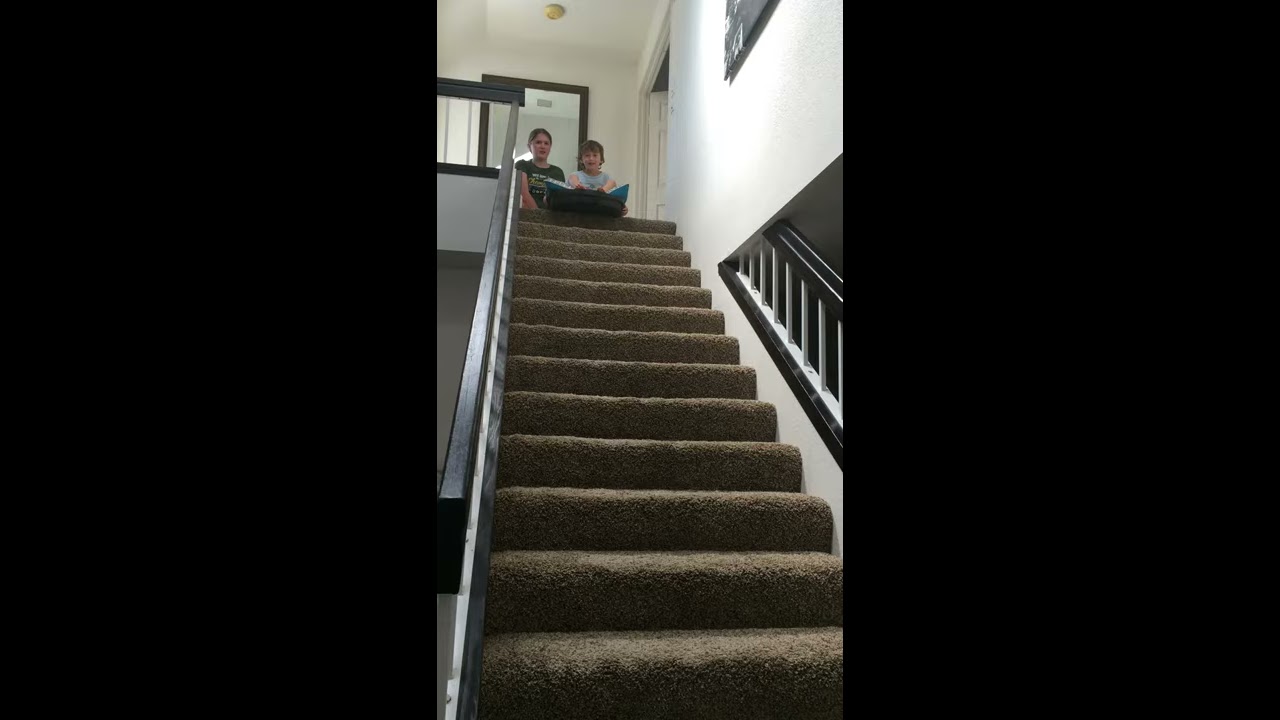The image depicts an indoor setting captured from the bottom of a centrally positioned staircase, looking upwards. The staircase is carpeted in brown and features handrails on both sides, with black top guards and white balusters. There are a total of 14 steps leading up to a doorway at the top. Positioned at the top of the stairs are two children, a girl and a younger boy. The girl, slightly older with brown hair pulled back and wearing a green t-shirt, stands beside the boy. The boy, who has shaggy hair and is donned in a light blue or gray shirt, sits on a makeshift sled, possibly a trash can lid or a piece of bubble wrap, with his legs in a V shape, appearing poised to sled down the staircase. The scene, devoid of any text, is set in a residential environment and captured in the afternoon, characterized by the colors black, brown, gray, green, light blue, and yellow.